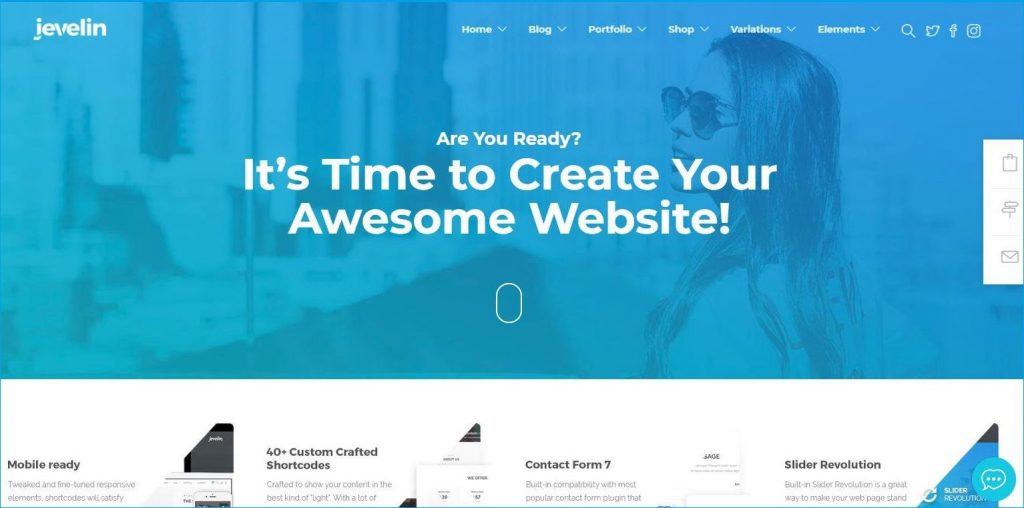The screenshot of the website displays the homepage of "Jevelin," with its name prominently positioned at the top left corner, stylized with a distinctive logo that features a slash through the letters 'J' and 'V'. In the top right section of the screen, a comprehensive navigation menu has several drop-down options labeled: Home, Blog, Portfolio, Shop, Variations, and Elements, each indicated by a downward-facing arrow.

Central to the image is a bold headline stating, "Are You Ready? It's time to create your awesome website." Below this, although partly obscured, text advertises key features such as "Mobile Ready, 40+ Custom Crafted Shortcodes, Contact Form 7, and Slider Revolution."

On the right side of the screen, a series of icons are visible, representing functions such as email, shopping bag, and a signpost, with a chat icon located at the bottom right. This indicates potential customer support or help option. 

The context suggests that Jevelin offers a platform designed to help users build highly customizable, professional websites with ease, emphasizing a variety of features that cater to mobile compatibility and numerous customization options. The site appears to be user-friendly and supportive for individuals or businesses seeking a ready-made yet flexible website solution.